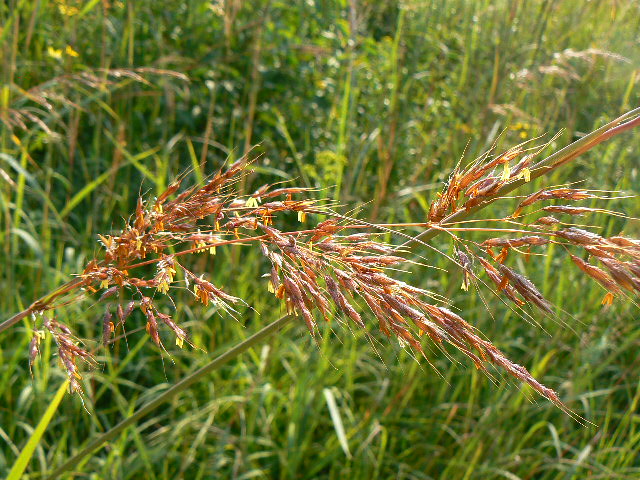The photo captures a lush, green field densely populated with tall grass and various weeds. Central to the image is a single branch of brown, wheat-like grass that stands in sharp focus, characterized by its long, hay-like strands and small pellet-like ends. Surrounding this focal point are diverse plant elements, including white and yellow weed flowers, contributing to the richness of the scene. The lighting suggests it was taken during the daytime, with sunlight streaming in from the top right, illuminating the vibrant greenery and creating reflections that indicate it is a sunny day. The setting appears to be outdoors in a possibly marshy area, suggesting a potential for wet, mucky ground underfoot, adding a sense of environmental immersion. All these elements together evoke the serene, natural atmosphere commonly experienced in the summertime.